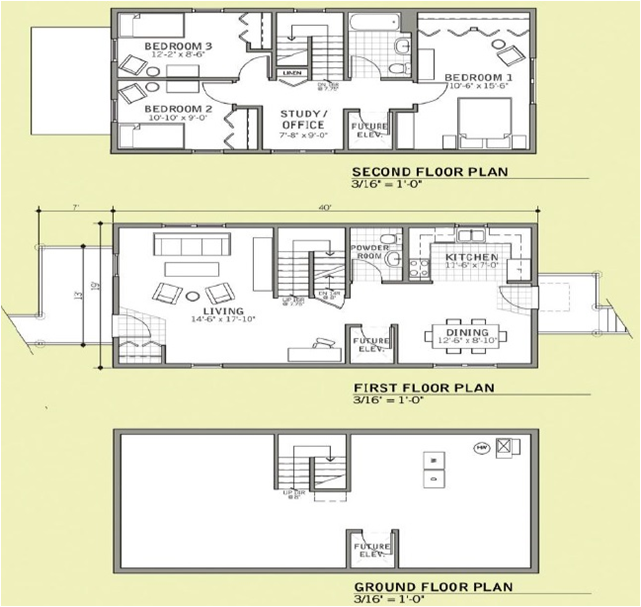This image showcases detailed architectural floor plans of a three-story building. There are three distinct rectangular sections in the image, each representing a different floor level. 

At the top is the second-floor plan, followed by the first-floor plan in the middle, and then the ground-floor plan at the bottom. Each floor plan features a horizontal black line beneath it with the notation "3/16 = 1-0" indicating the scale of the drawings.

The second-floor plan depicts a layout with three bedrooms: Bedroom 1 on the right, and Bedrooms 2 and 3 on the left, arranged one above the other. Centrally located, there's a study or office space. Adjacent to this area, an unlabeled bathroom can be identified by the presence of tile flooring, a tub, a sink, and a toilet. Additionally, there is a diagram of a staircase with an arrow pointing downwards, indicating its direction.

The first-floor plan offers a detailed view of a kitchen that opens into a dining room, with specific measurements given for these areas. Next to the kitchen, there is a powder room. Beyond the dining area, a large living room is depicted, occupying a substantial portion of this floor.

Lastly, the ground-floor plan is relatively simple, featuring only a set of stairs leading upwards.

This comprehensive and detailed image provides an insightful glimpse into the spatial arrangement and design of the building's three floors.